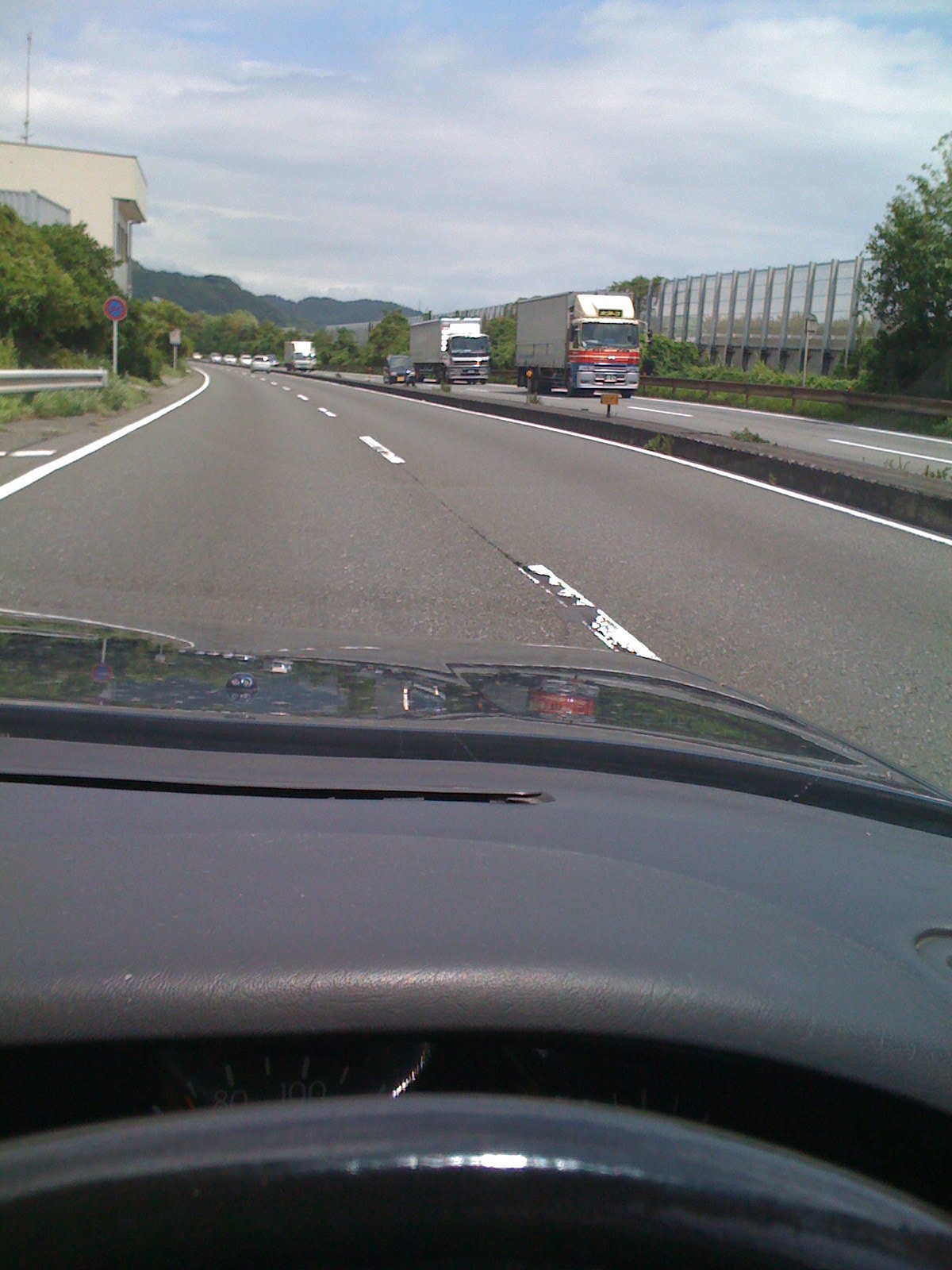A detailed image captured from inside a car traveling on a highway showcases multiple intriguing elements. The prominent black dashboard contrasts with the slight glimpse of the black hood and steering wheel. Partial dashboard controls displaying numbers like 80 and 100 are partially visible, though not entirely clear. An unusual orange reflection on the hood adds a touch of mystery, perhaps hinting at the surrounding traffic.

The highway, marked with white dividing lines, features an unconventional traffic pattern. Vehicles traveling in the opposite direction appear on the right side of the road — a setup different from typical left-hand driving scenarios. The opposing traffic includes a mix of large trucks and cars. To the right, the scene includes visible buildings and trees, while to the left, there are more buildings and additional foliage, contributing to a somewhat disorienting yet intriguing view of the road.